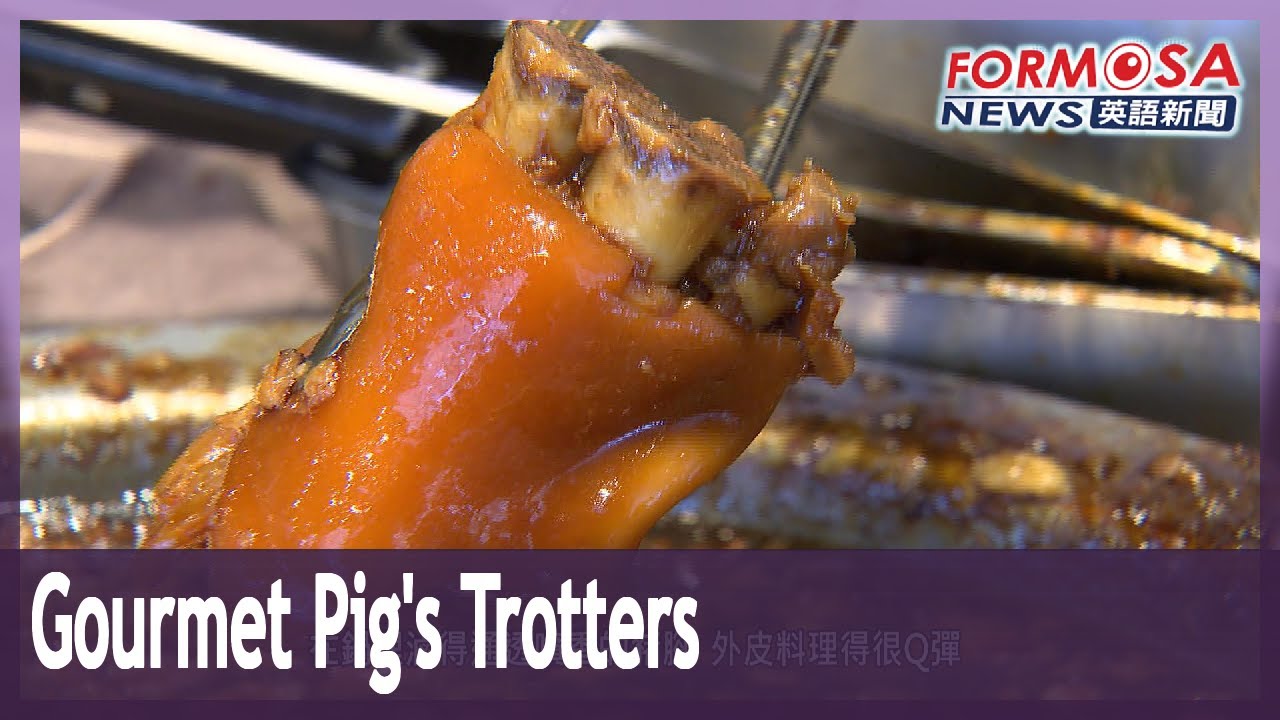The image depicts a broadcast advertisement for Gourmet Pig's Trotters. Dominating the image is a close-up photograph of a cooked pig's foot, displaying a rich golden-brown, almost orange hue, suggestive of being well-cooked. The foot, with visible bones extending from the cut end, appears shiny and slightly sticky, as if pulled from a broth or batter, and is held by a pair of tongs. The setting seems to be a stainless steel kitchen or the interior of a large grill, providing a professional culinary backdrop. In the bottom quarter of the image, a blue overlay features white text reading "Gourmet Pig's Trotters" along with Chinese characters. The upper right corner of the image displays the news channel's name, "Formosa News," followed by several Asian characters, possibly Japanese or Chinese, indicating the likely location of the broadcast.